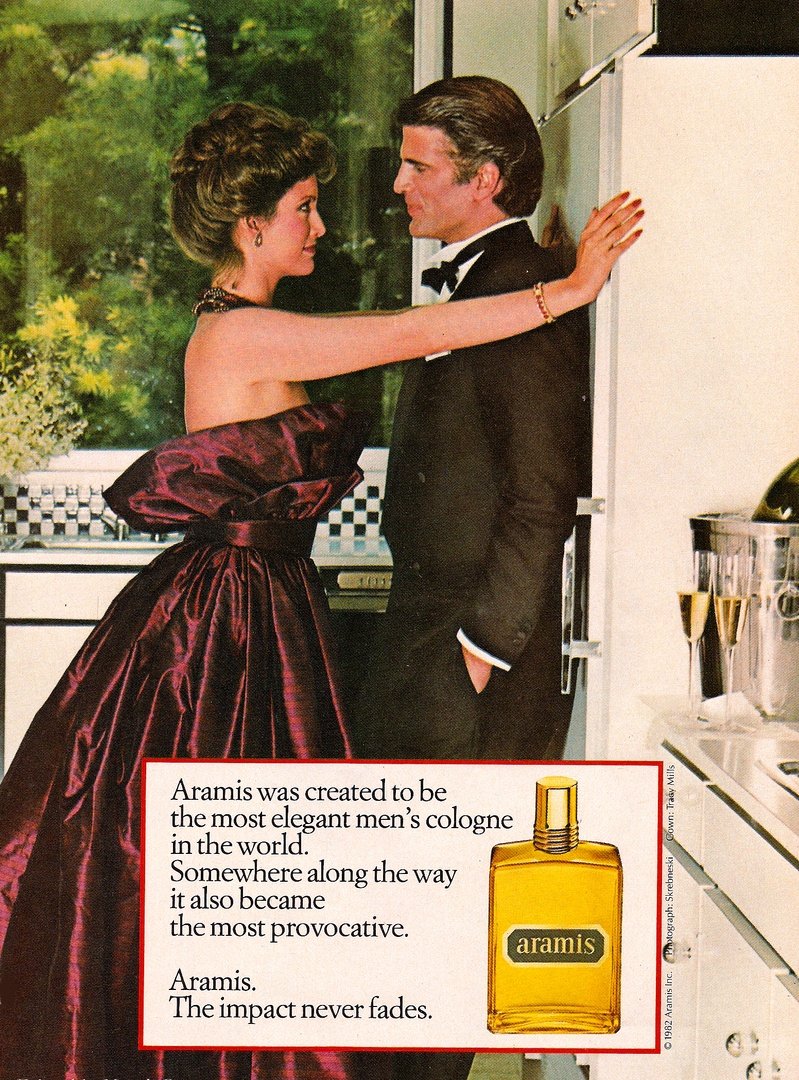The image is a vintage magazine advertisement for Aramis cologne, prominently featuring a golden bottle labeled "Aramis" (spelled A-R-A-M-I-S). At the bottom of the ad, within a white rectangle framed in red, the text reads: "Aramis was created to be the most elegant men's cologne in the world. Somewhere along the way it also became the most provocative. Aramis. The impact never fades," all in black font.

In the scene, a sophisticated man with brown hair, dressed in a classic black-and-white tuxedo, leans against a white refrigerator. He is being approached intimately by a woman with brown hair styled up, adorned with earrings. She is wearing an elegant, shiny evening gown, varying between red, magenta, mauve, and burgundy shades, with a fluffy texture. Her arms are raised, pinning the man against the fridge, creating an intense and provocative atmosphere. 

The setting appears to be a stylish kitchen, with visible details including a window revealing green trees, wine glasses, a bottle of wine, pots, a sink, and a dishwasher. The portrayal suggests a glamorous and intimate domestic scene, amplified by the presence of luxurious elements and the alluring interaction between the man and woman.